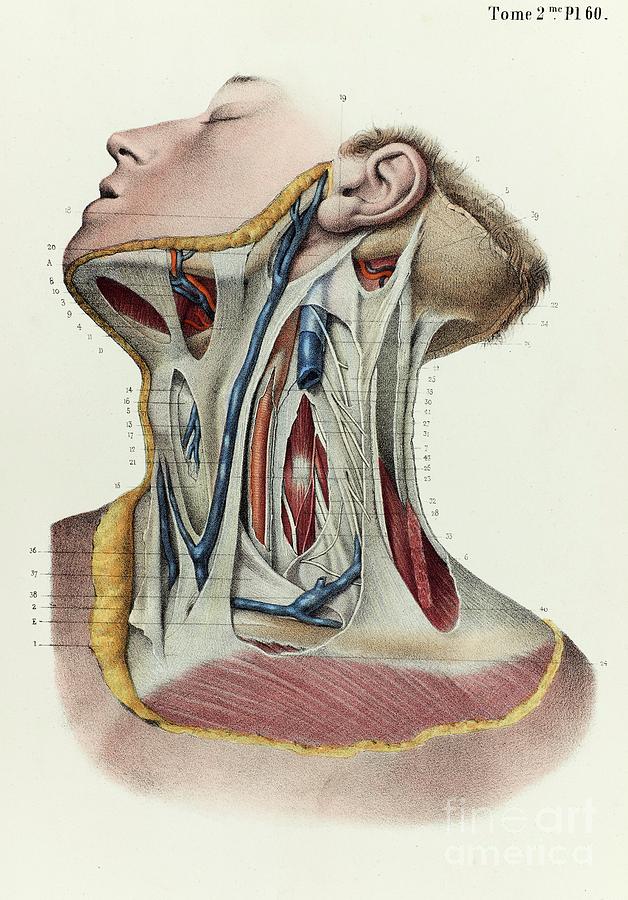This detailed scientific illustration, likely hand-drawn with colored pencils, depicts a dissection of a human neck, showcasing the musculature, veins, and arteries. The image presents the left side of a light-skinned figure, with the head tilted up and to the right, revealing a clear profile from the shoulder up to the eyebrow. The top part of the skull is absent, exposing the underlying anatomical structures. The face retains its skin, while the neck and lower jaw reveal the intricate network of muscles, tendons, arteries, and veins, meticulously labeled with various numbers and letters. These labels, although numerous (ranging from 20 to 40), lack accompanying descriptions. The background of the image is beige, and in the top corner, the text "Tome 2 MEP 160" is visible, suggesting a reference to a specific volume or section, enhancing its appearance as a detailed excerpt from a scientific journal or textbook.